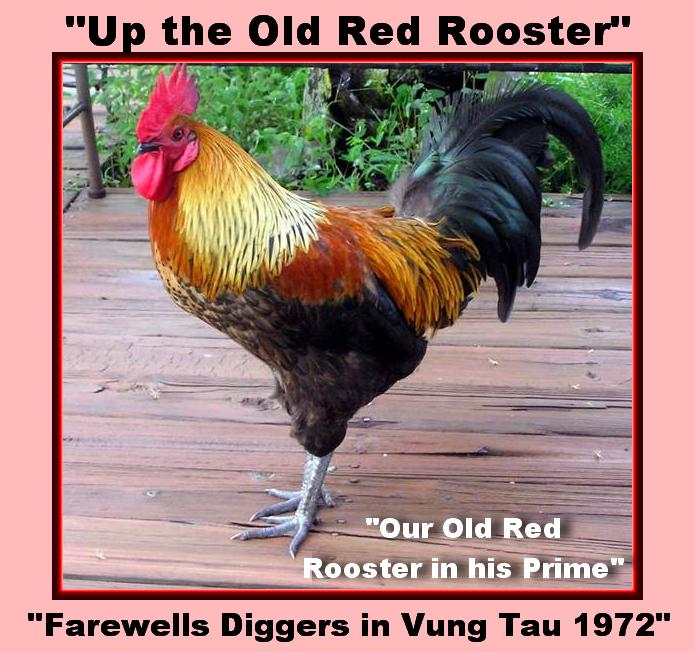This image features a beautifully detailed color photograph of a large rooster with striking reddish-brown plumage, a bright red comb and waddle, bluish-gray feet, and greenish tail feathers. The rooster is prominently placed in the center, standing on a wooden slatted surface, likely a patio, with some vegetation visible in the background. The photograph is in a square format and is set against a pinkish-reddish background. The image is surrounded by a digital or computer-generated border that features a black outline with an inner red outline. At the top of this border, bold black text within quotation marks reads, "Up the Old Red Rooster," while the bottom displays, "Farewells, Diggers in Vung Tau, 1972," also in bold black text. Superimposed in white text in the bottom right corner of the photo, it says, "Our Old Red Rooster in His Prime." The rooster is turned slightly to the side, looking up towards the viewer, showcasing its impressive feathers and presence. The overall style combines color photography with a graphic design and typography overlay, creating a vivid and nostalgic tribute.